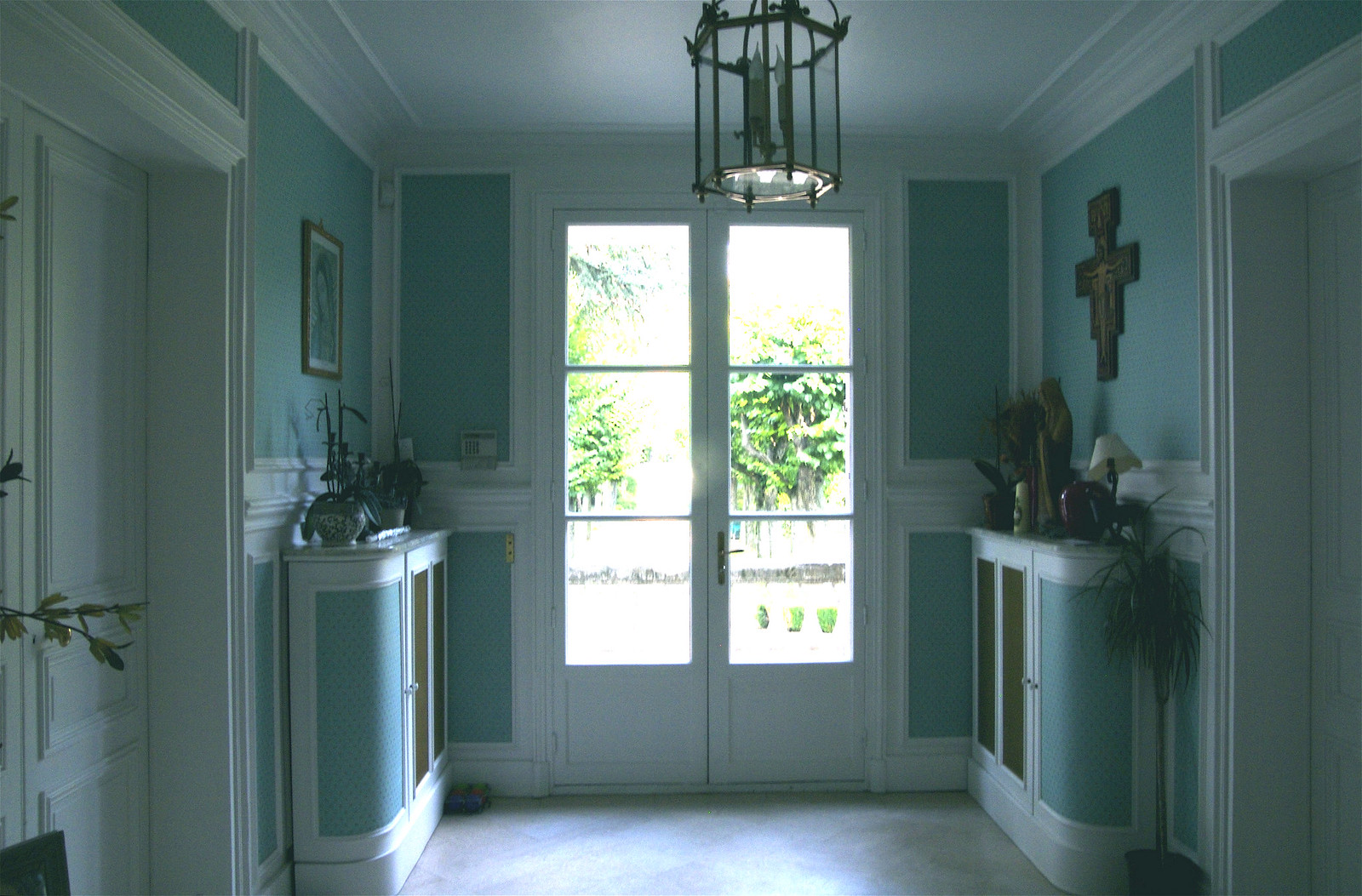The image showcases the interior hallway of a fancy beach house with seafoam green walls. Through the hallway, a picturesque view of lush green shrubbery and trees can be seen outside. Inside the house, there are green plants on both sides; a prominent plant with abundant leaves is on the right, while another plant adorns the left. The ceiling features a lantern, adding to the elegant decor. The walls are decorated with artwork, possibly of a religious nature, enhancing the house's sophisticated ambiance. The overall impression is of an old yet opulent beach house with meticulously maintained greenery both inside and out.